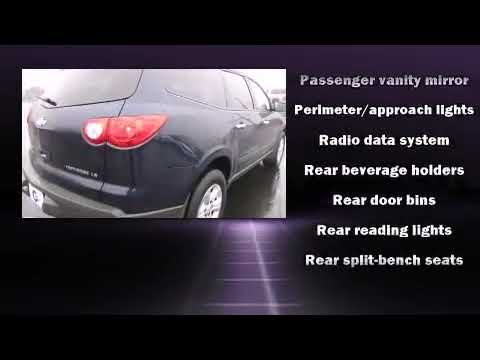The image depicts the rear view of a dark blue or black van with red taillights and a rear windshield wiper, framed within a small square. The overall photo has black borders on the top and bottom, while the central background features a deep purple color. Illuminated by white light in the center, the right side of the purple section contains white text listing features such as "passenger vanity mirror, perimeter approach lights, radio data system, rear beverage holders, rear door bins, rear reading lights, rear split bench seats." The scene features a mix of light and shadows, and although the vehicle's brand and model remain indistinct, the image effectively highlights specific characteristics and ambient lighting.